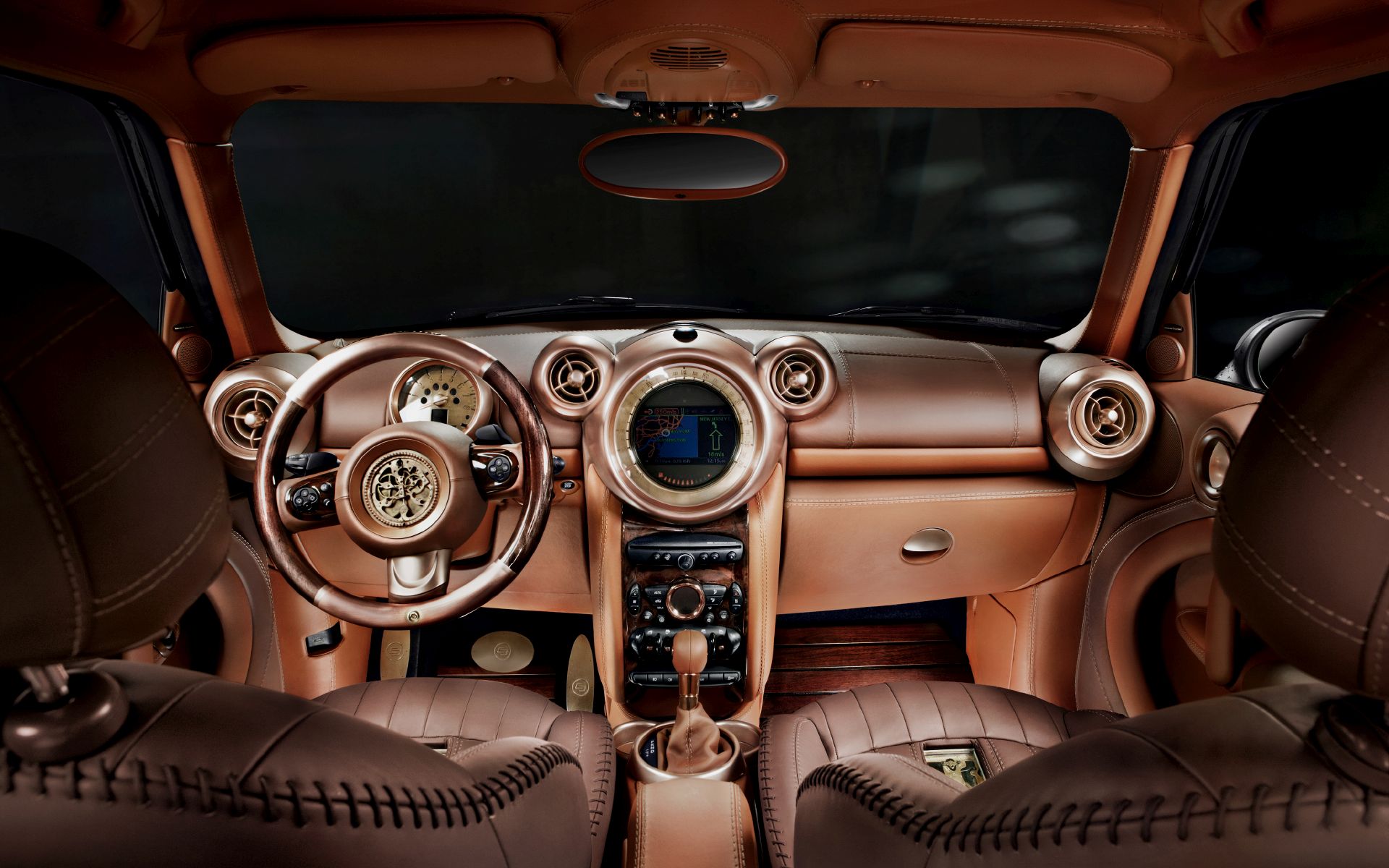This highly stylized photo captures the luxurious interior of a modern car, as seen from the middle of the back seat. The interior exhibits a rich, dark brown and gold color scheme with diverse shades of brown throughout. The seats, half-visible in the shot, are adorned with deep, intricate baseball-like hand stitching, adding to the opulent feel. The floorboards are intriguingly made of wood, a unique and distinguished touch.

In front, the dashboard and the center console feature high-end leather or similarly premium materials, emphasizing the car's sophistication. The steering wheel, also in gold, stands out with its three spokes connecting to a central part that holds a crest, accentuating its distinctly stylish and possibly steampunk design. Below, we notice a manual gear shift, hinting at a four or five-speed transmission, along with visible gas, brake, and clutch pedals.

The center console extends upward to a navigation system integrated into the dash. The air conditioning vents, round and somewhat vintage in style, continue the circular motif found throughout the car's design. Above, the windshield stretches out, flanked by two sun visors, and showcases an oval rearview mirror with black trim. Outside, the surroundings are dark and indiscernible through the tinted windows, directing attention back to the sumptuous and futuristic car interior.